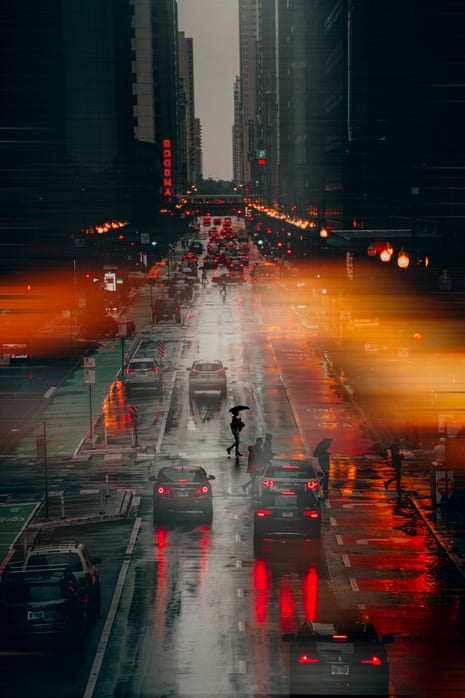This is a photograph of a bustling city street scene at nighttime, characterized by a primarily black and gray palette accentuated by vivid red and orange lights. The image showcases a straight, wet road lined with towering skyscrapers on both sides, leading into the distance. Cars are prominent on the rain-slicked road, with many stopped in traffic and displaying activated brake lights. Pedestrians, some holding umbrellas, are seen crossing the street, their silhouettes and the reflections of the city lights creating a hazy blur due to the rain. The vivid colors from street lights, traffic lights, and car lights punctuate the scene, heightening the overall contrast and adding a dynamic element to the photograph's otherwise dark and subdued tones.